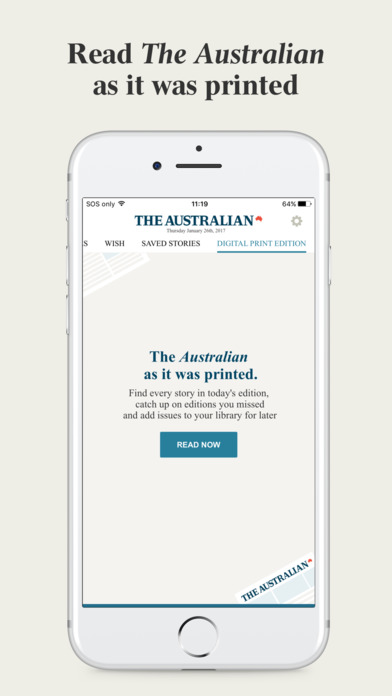The image features a white cell phone against a very light green background. The advertisement text on this background is formatted in two lines, positioned with two spaces from the top and two to three spaces to the right from the left side. The first line reads "Read The Australian," followed by "as it was printed."

Below this text is a picture of the white cell phone. On the phone's screen, the same phrase, "The Australian," appears in larger, center-justified font. Notably, in the top-left corner of the phone screen, it displays "SOS Only" next to a Wi-Fi icon, indicating a lack of cellular signal. The time shown on the phone is 11:19, and the battery is at 64%.

In the center of the screen, "The Australian as it was printed" is prominently displayed once more. Beneath this phrase, there is a short blurb, followed by a "Read Now" button, suggesting immediate access to the content.